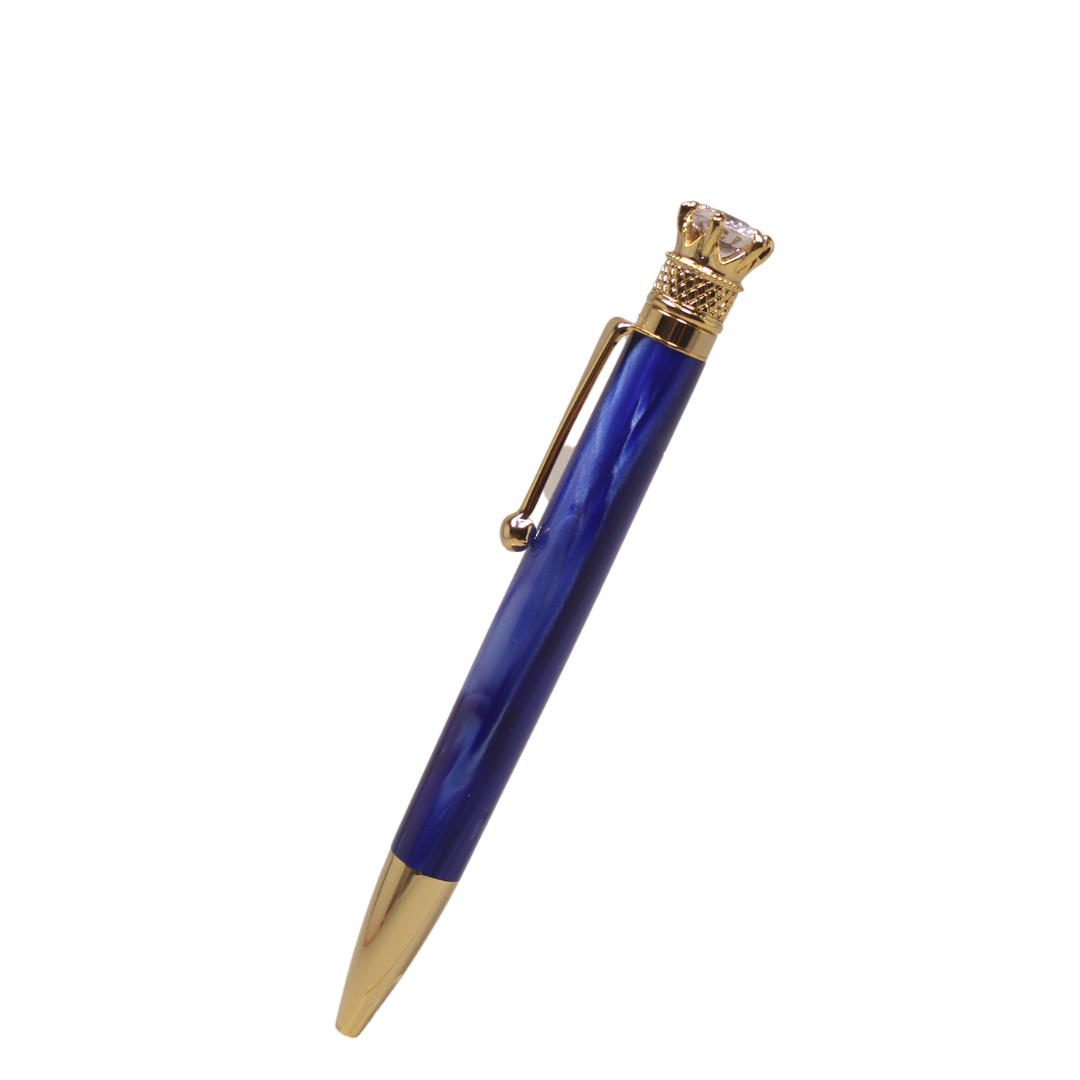The image depicts a short, fancy pen positioned diagonally from the upper right to the lower left corner against a pure white background. The pen's body has a smooth, shiny finish in shades of navy and royal blue, with subtle lighter streaks running through it, giving it an elegant appearance. It features a golden nib and a matching gold end cap where the ink is released. A goldish pen clip, adorned with a little ball at the end, is attached to the pen, allowing it to be clipped onto a pocket. At the very top, where one would typically find an eraser on a pencil, sits a large, clear stone resembling a diamond, held in place by gold prongs. The overall look of the pen is polished, luxurious, and contemporary, suggesting it is a high-end writing instrument. The clean and simple background further accentuates the pen's sophisticated design.